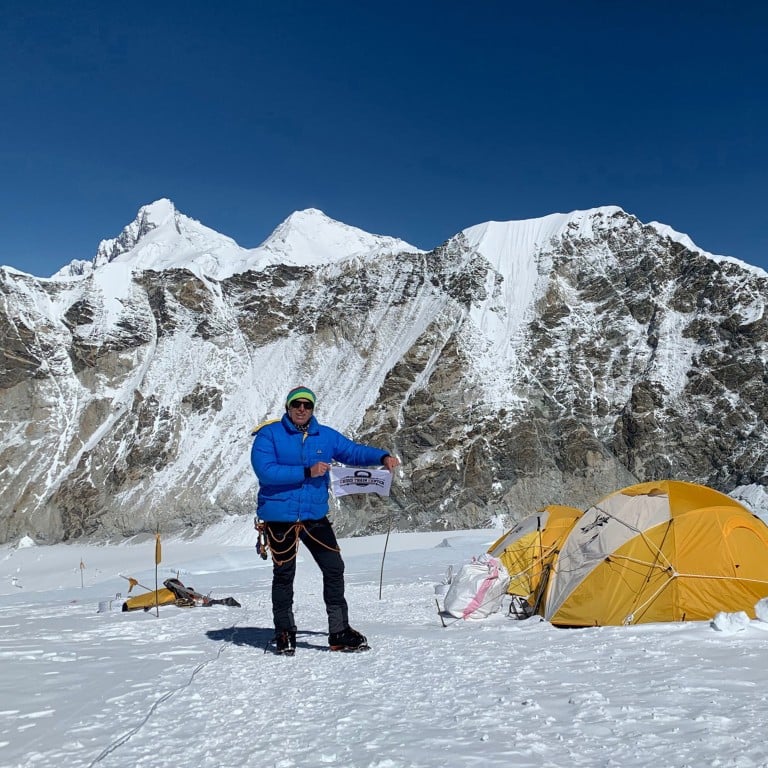In this photograph, an older man is standing proudly on a hard-packed snowy surface, appearing as though he has reached the summit of a mountain. He is dressed for very cold weather with black snow pants, black shoes equipped with crampons, and a blue jacket. He also sports a beanie hat that features two shades of green and a pair of sunglasses, likely to protect against snow glare. Hanging from his jacket is essential mountain climbing equipment, with ropes for safety. In his hands, he holds a small sign or flag, although the text on it is unreadable.

Surrounding him are two small dome tents, colored gold and white, with various supplies scattered nearby. Beyond the immediate camping area, towering snowy mountains dominate the backdrop beneath a mostly clear sky. The image's composition suggests it could serve as a keepsake, for social media, or even for a magazine, capturing the essence of the man's adventurous spirit and the stark, beautiful environment he has conquered.